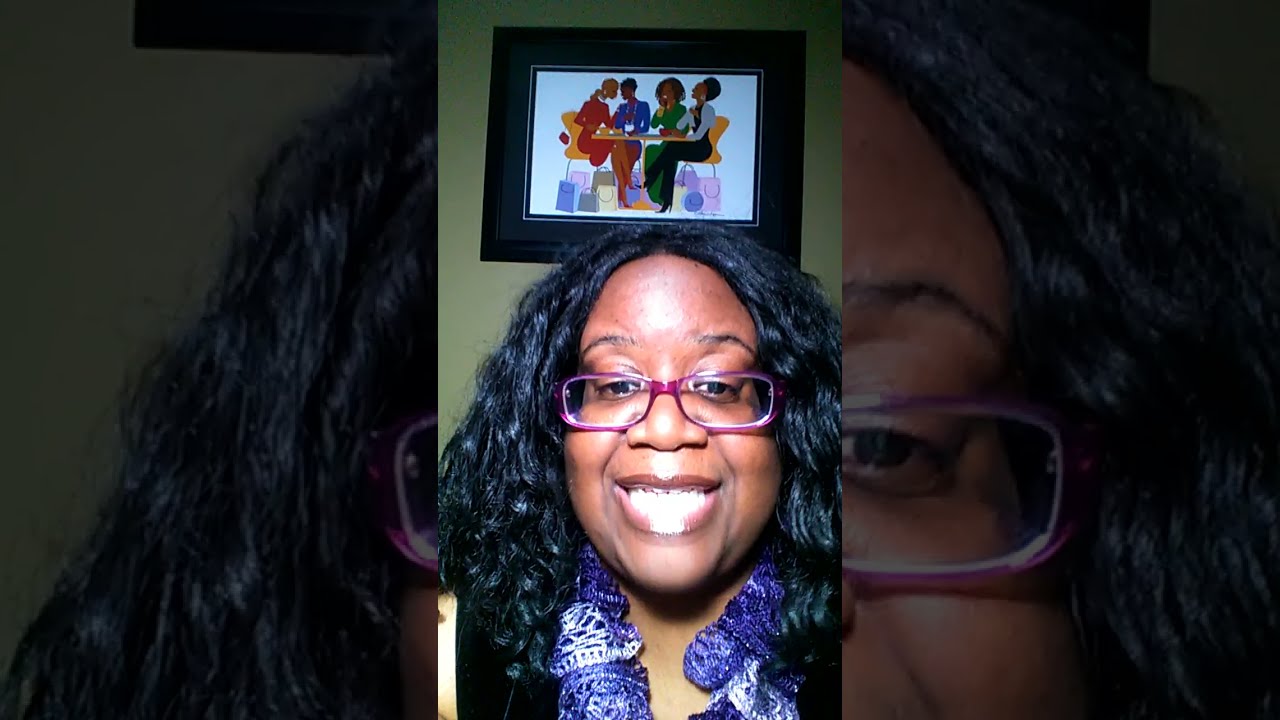In this portrait-oriented image, a dark-skinned woman with shoulder-length, wavy black hair and light pink lips smiles brightly, revealing both her upper and lower teeth. She is adorned with vibrant rectangle-shaped fuchsia glasses and wears a bluish and purple scarf around her neck, paired with a black top. The setting appears to be indoors, likely her home, with a green wall serving as the background.

A prominent feature of the image is the artwork hanging above her head, showcasing four dark-skinned women seated at an orange table, each dressed in different colors: a red dress, a blue dress, a green dress, and a black and white suit ensemble. The women in the artwork seem joyful, possibly laughing, and have various colored bags, including blue, white, cream, brown, and purple, beneath their chairs and table. The picture frame is black with a black outline.

The image composition includes a detailed central portrait of the woman, flanked by grayed-out, close-up versions of her eyes and part of her face, adding depth and context to her expression within the dimly lit setting.